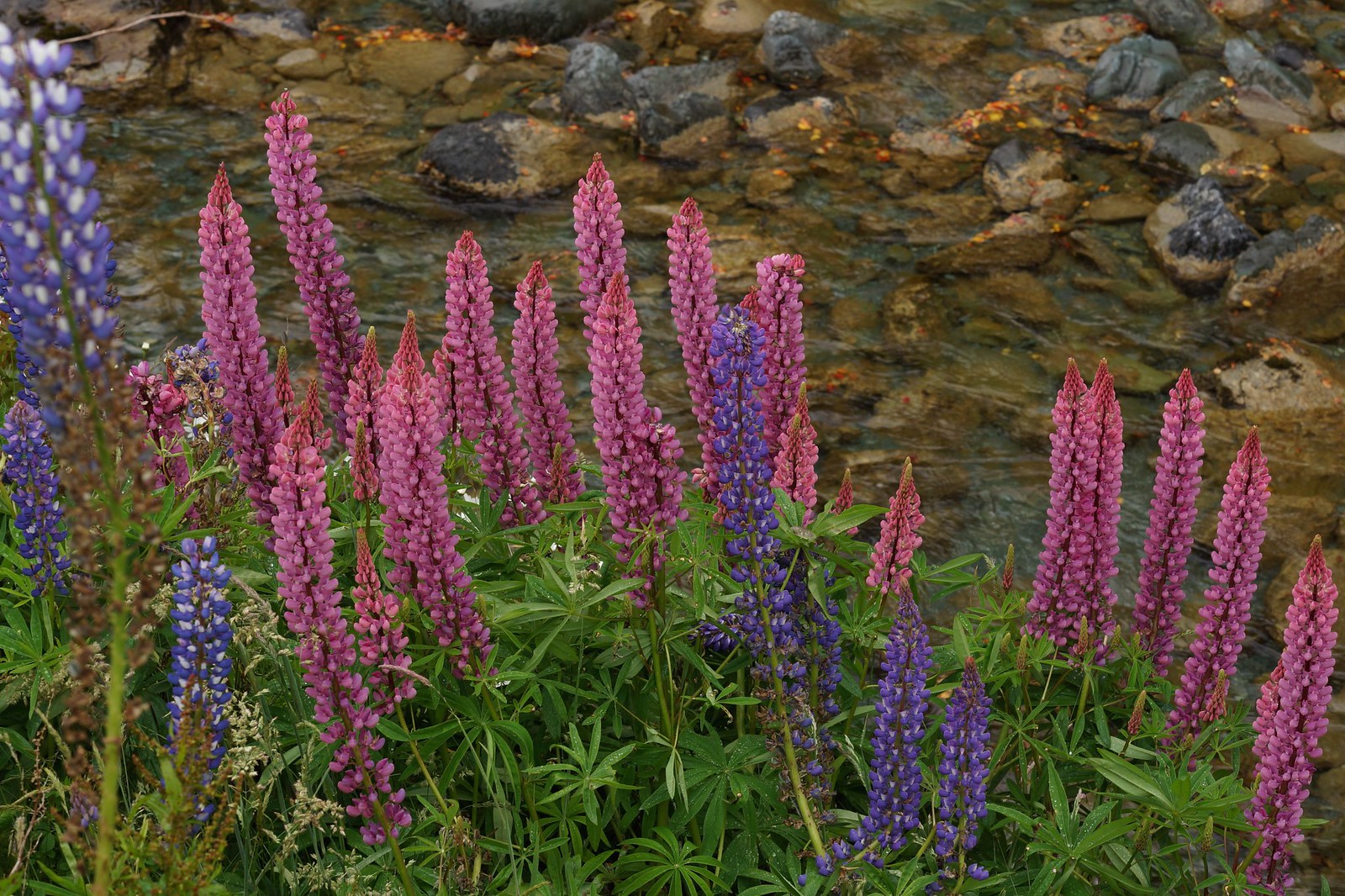The color photograph is an outdoor close-up capturing a vivid display of tall, tower-like flowers and bright green grasses set against a backdrop of large stones. The flowers, predominantly dark pink and medium purple, are not mixed; each stem supports blossoms of a single color. Several flower stems, which may be lupins, rise straight up like towers, with blooms and tiny flowers sequentially aligned up the stalks. The green grasses at the bottom of the image sport long, slender, pointy leaves, some of which are star-shaped with more than five points. The background features large rocks in shades of brown, dark gray, and black. The image is bright and clear, taken in natural outdoor light, showcasing the vibrant colors and details of the flowers and grasses with high clarity and quality.